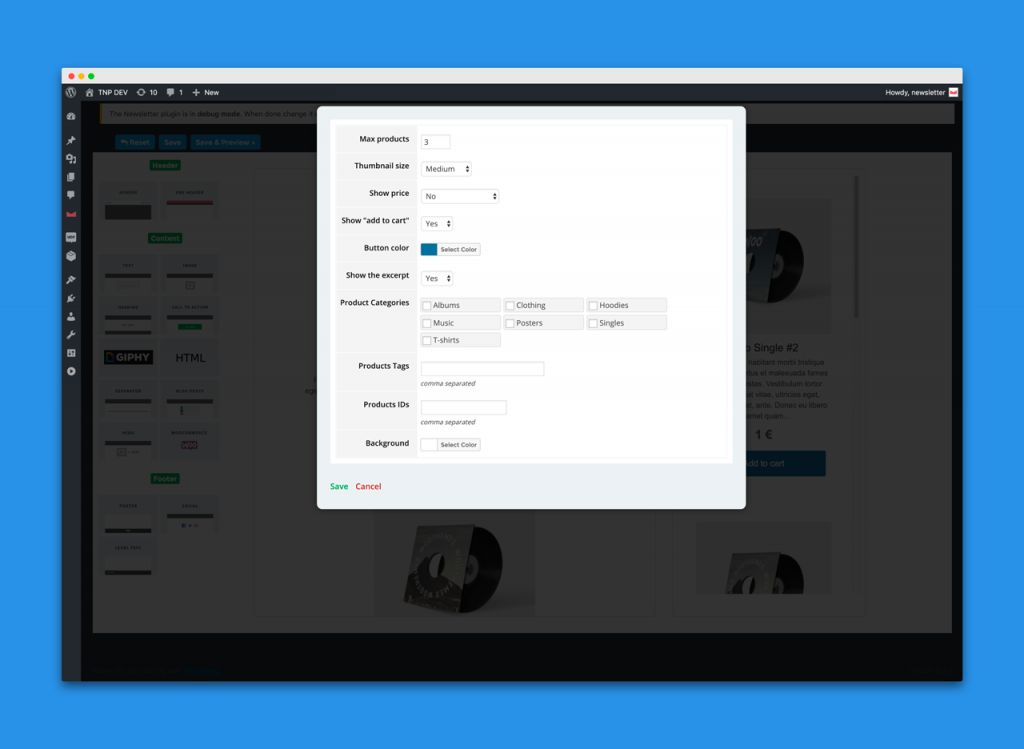The image displays a computer screen with a central pop-up window. Surrounding the screen is a light blue background on all sides—top, bottom, right, and left. 

In the top left corner of the screen, there are three control dots: a red dot, a yellow dot in the middle, and a green dot on the far right. Below these dots, a series of small tabs and icons are arranged vertically along the left side of the screen, extending from the top to about the center.

The screen appears to have a holographic gray tint due to the activation of the pop-up window, slightly dimming the visible content in the background. The pop-up itself is centered and features a series of options. Categories are listed on the left side of the pop-up in black text, with corresponding options on the right.

At the top left of the screen, three small light blue rectangles are discernible. Below these, there is a green rectangle. Further down, within the pop-up, categories are again listed on the left, followed by four options positioned centrally: 

1. The first option is obscured.
2. The second option is partially visible and features a blue rectangle beneath it.
3. The third and fourth options contain images within gray squares.